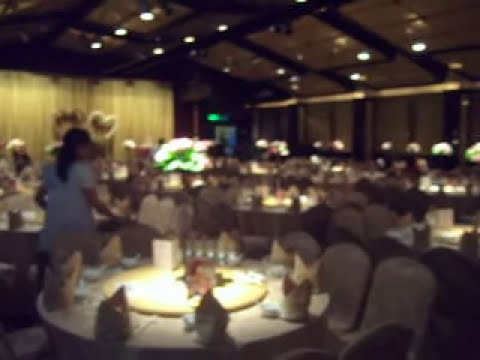The image depicts a large, dimly-lit event space, possibly a Chinese restaurant or catering hall, with high ceilings and beige walls. The foreground features a large round table with seats surrounding it, each set with a napkin folded in a manner that almost resembles a hat, and place mats. At the center of the table, there is a rotating platform typical of Chinese dining setups, allowing guests to share food family-style. There are multiple tables scattered throughout the space, all similarly arranged with tablecloths and decorative napkins. Some tables also feature flowers as part of their centerpiece decoration. People are seen seated and moving around the tables, hinting at a lively atmosphere. A stage is visible to the left, adorned with heart-shaped flower arrangements, suggesting that this could be a wedding or another celebratory event. The overall color scheme includes shades of white, yellow, green, tan, brown, black, and blue. Despite the blur, the image captures the essence of a festive gathering with lights and possibly candles enhancing the ambiance.